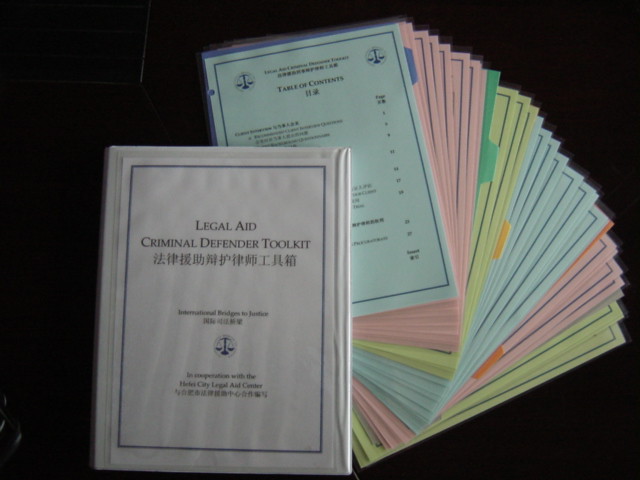The photo captures a collection of pamphlets titled "Legal Aid Criminal Defender Toolkit," displayed on a table covered with a black cloth. The centerpiece is a white document prominently featuring the title in black text, accompanied by Asian characters and an icon of the scales of justice. Surrounding this central pamphlet are numerous other documents, organized in a fan-like arrangement. These additional pamphlets, varying in colors such as light blue, yellow, pink, white, and green, each feature their own headings and decorative icons, including scales of justice. The layout provides a sense of organization and emphasis on the contents of the toolkit, though the text on some materials is obscured by overlapping pages, making it difficult to discern specific details from the distance of the photograph.